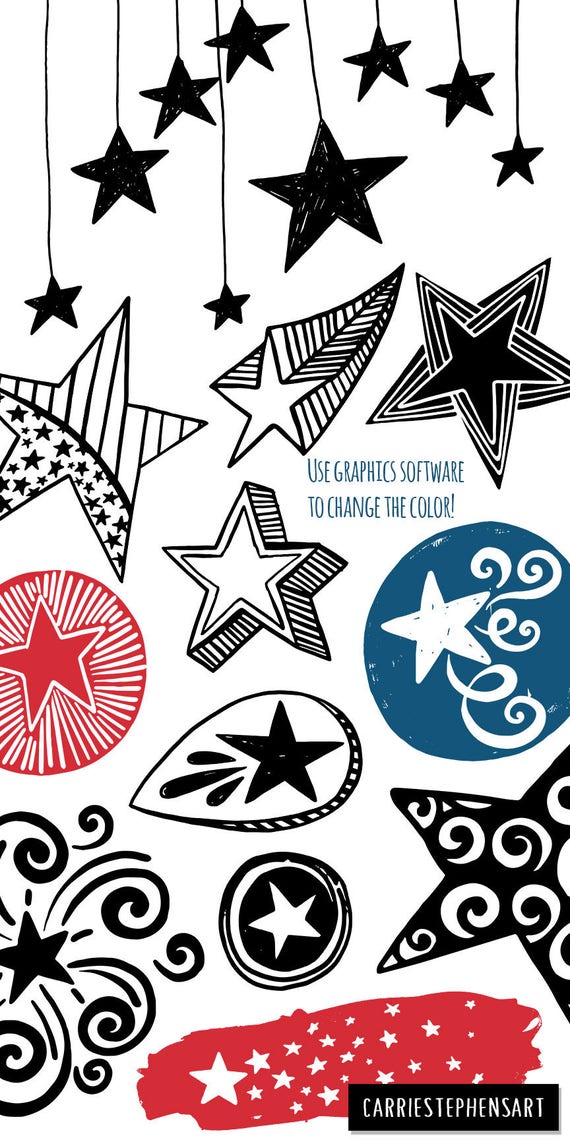This promotional product photo, titled "Carrie Stevens Art," showcases a collection of star-themed graphic designs in a predominantly black-and-white palette with accents of red and blue. At the top, black stars hang from strings, creating a whimsical backdrop. A layered row of black-and-white stars, each uniquely detailed, adds depth and texture to the composition. Among these designs are instructions in text, "Use graphics software to change the color!"

Central features include a striking red circle with a white star, from which white lines radiate outward, and a blue circle encasing a white star, adorned with elegant swirls and curlicues. Another notable element is a teardrop-shaped design with a star inside, accented by black droplets. Additionally, a red swatch, reminiscent of a paintbrush stroke, is filled with white stars. This intricate blend of star shapes and color splashes highlights the versatility and creativity of graphic art. The image is signed at the bottom in a black bar with white letters by the artist, Carrie Stevens.